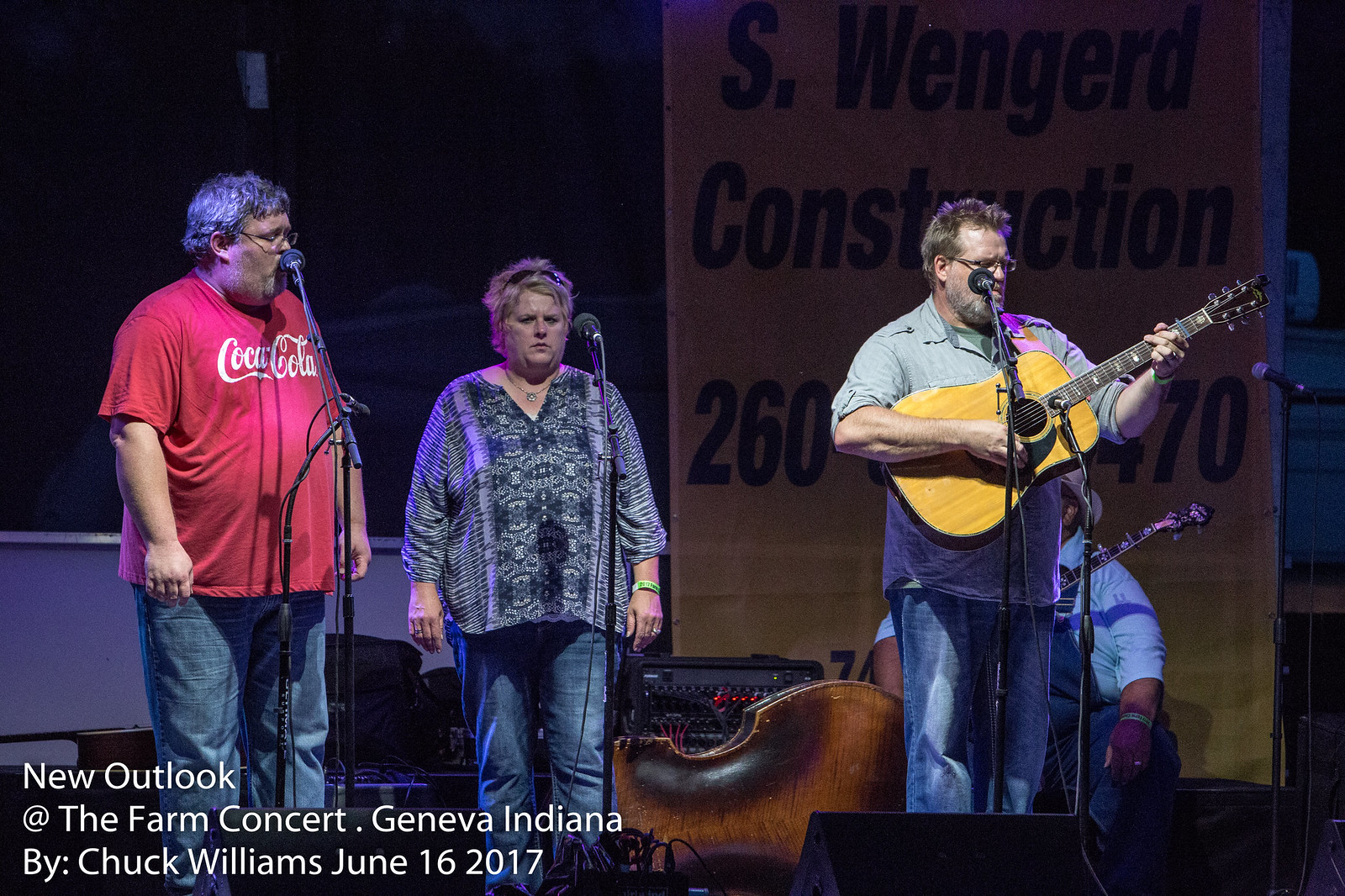This detailed photograph captures four musicians on stage during a nighttime performance at the "New Outlook at the Farm Concert" in Geneva, Indiana, taken by Chuck Williams on June 26, 2017. From left to right, the first musician is a middle-aged man wearing a red Coca-Cola t-shirt with white lettering, paired with blue jeans. He stands at a microphone, appearing to sing. The second musician is a woman with a short haircut and an expressive, somewhat stern face. She is dressed in a loose-fitting purple and black blouse and blue jeans, sporting a green wristband, and also stands at a microphone. To her right, the third musician, a man with glasses and short brown hair, is playing an acoustic guitar. He wears a green shirt and blue jeans and holds the guitar up to a microphone. Partially obscured behind him is a fourth, larger man, dressed in a light blue shirt and dark blue overalls, holding another string instrument, possibly a banjo. A bass violin lies on its side in front of the musicians. The stage backdrop features a large yellow banner with the text "S. Wengerd Construction" visible at the top, though the lower part of the banner is blocked by the performers. The overall scene is framed by the night, giving the background a solid black appearance, save for a brown banner descending from the upper right.